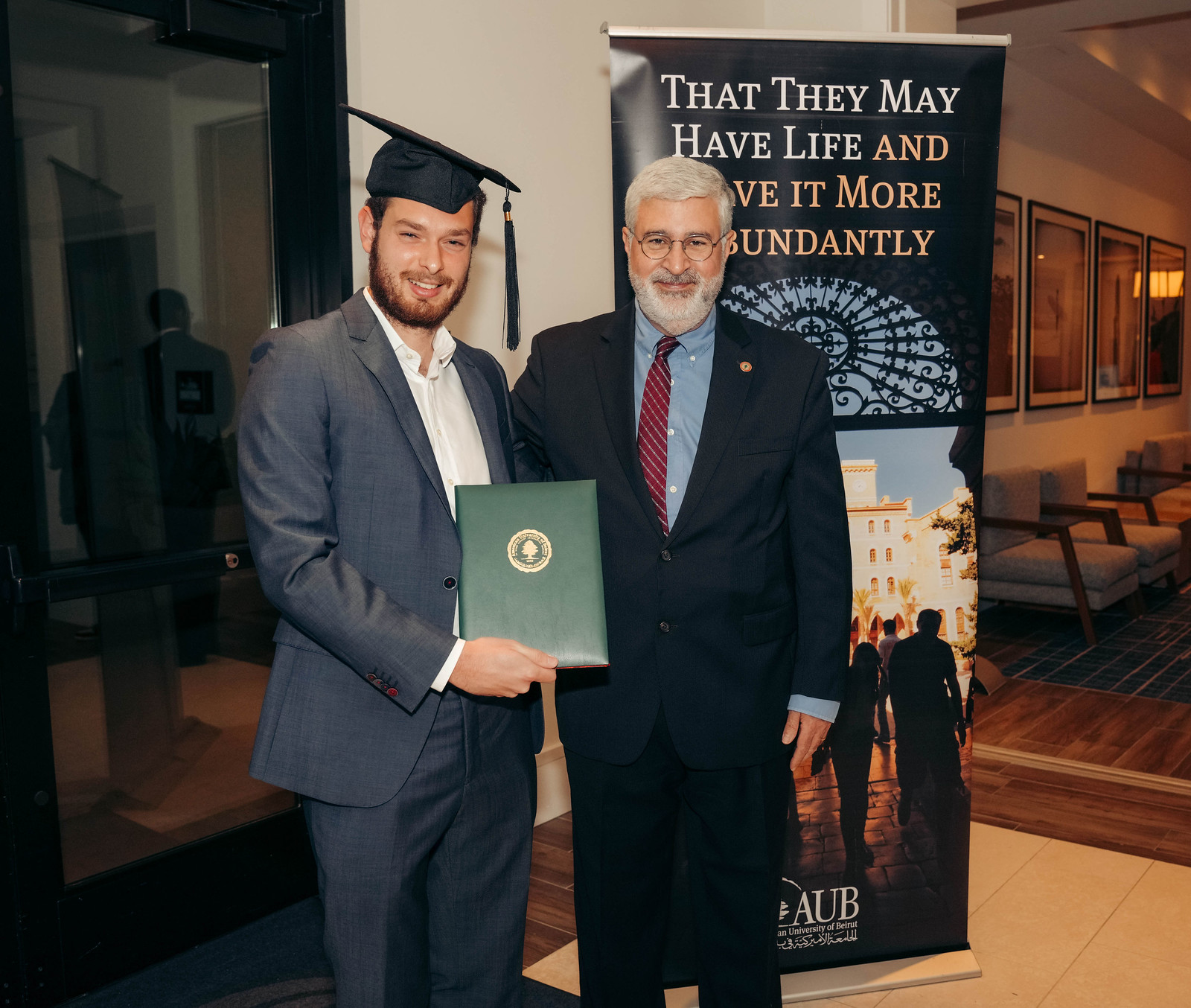This image features a younger man standing on the left, dressed in a grey suit with a white button-up shirt and a graduation cap with a black tassel perched on his head. He holds a green graduation booklet adorned with a gold emblem. Beside him stands an older man, likely his father, attired in a deep blue suit, a light blue shirt, and a red tie. The older man has grey hair, a grey beard, and wears glasses. Behind them is a partially visible banner proclaiming "that they may have life and have it more abundantly," along with an abbreviation "AUB" indicating the school. The background includes chairs resembling those found in a waiting room, and various paintings lined up on the walls. Additionally, there's a reflection of the two men in a glass door on the left side of the photograph, and the floor appears to be either tiled or wooden.